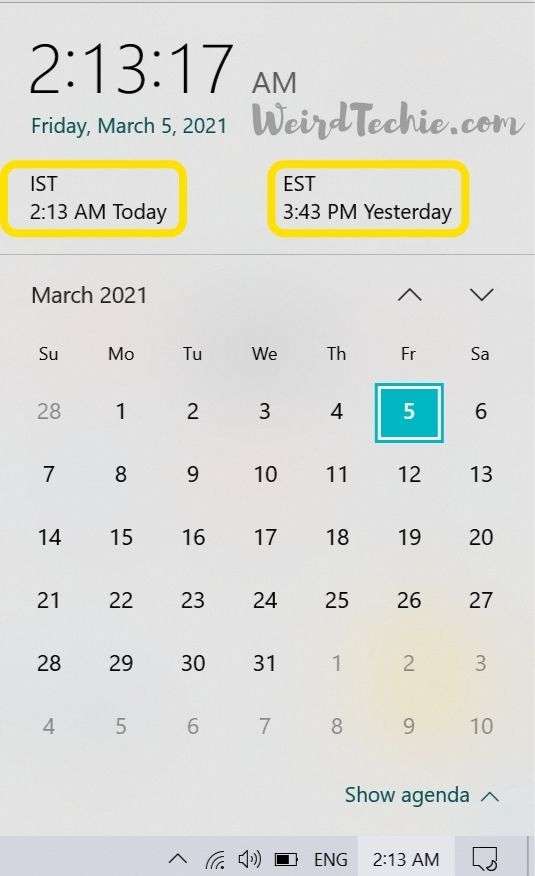This image displays a detailed screenshot of a calendar from weirdtechie.com. The calendar is set to Friday, March 5, 2021. The date "IST 2:30 AM" is highlighted in yellow, indicating an event or important note for that specific time. Adjacent to it is the equivalent time in Eastern Time (ET), marked as 3:43 PM.

The calendar layout covers the entire month of March 2021, including all days from Sunday through Saturday. It begins with the last day of February (28th) as the first day and runs sequentially through March, denoted up to the 31st. The currently highlighted date is March 5th, aligning with the present day.

At the bottom of the screenshot, there are additional utilities visible: a show agenda function for managing meeting notes, battery life indicator, volume control, language set to English, and the current time displayed as 2:13:00 AM, with hours, minutes, and seconds specifically noted.

The website's URL, weirdtechie.com, is mentioned prominently, indicating its source.